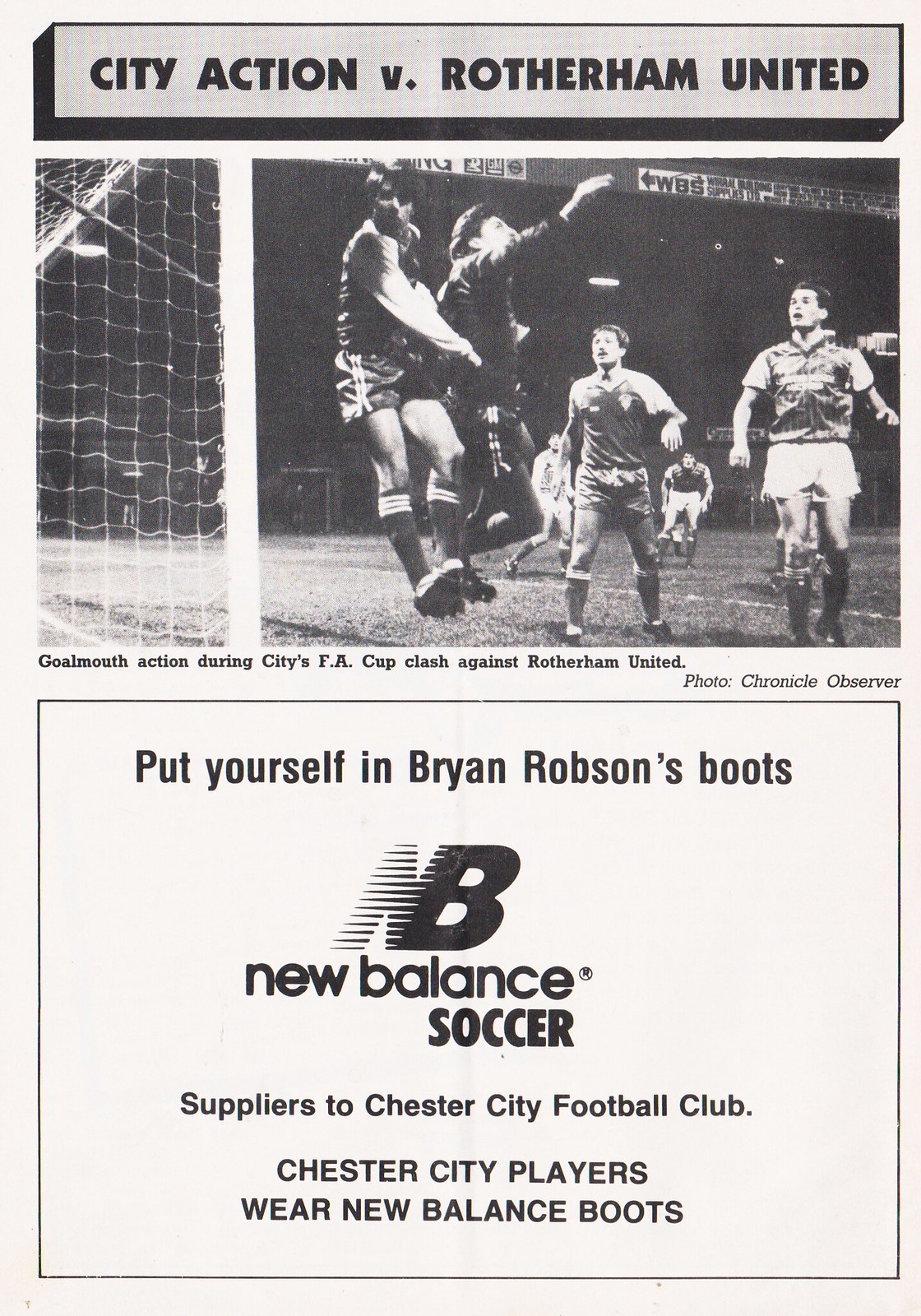This magazine page features a vintage aesthetic with an aged white background complemented by a subtle grey border along the top. The topmost part of the page displays the headline "City Action v. Rotterdam United" in bold black font. Below this headline, a black and white photograph captures a dynamic moment from a soccer match. The image shows a cluster of soccer players near the goal during an intense action sequence. On the left, two players are airborne, their feet entirely off the ground as they compete for the ball. Behind them, two more players stand with their mouths agape, seemingly in shock at the unfolding scene.

Beneath the photo, a caption in black text reads, "Golmuth Action during City's FA Cup clash against Rotterdam United, Photo Chronicle Observer." Directly below this caption is an advertisement bordered by a thin black frame, keeping with the vintage aesthetic by mirroring the same white background. The ad beckons readers with the phrase, "Put Yourself in Brian Robson's Boots," followed by the recognizable New Balance logo. Additional text informs, "New Balance Soccer: Suppliers to Chester City Football Club. Chester City players wear New Balance boots."